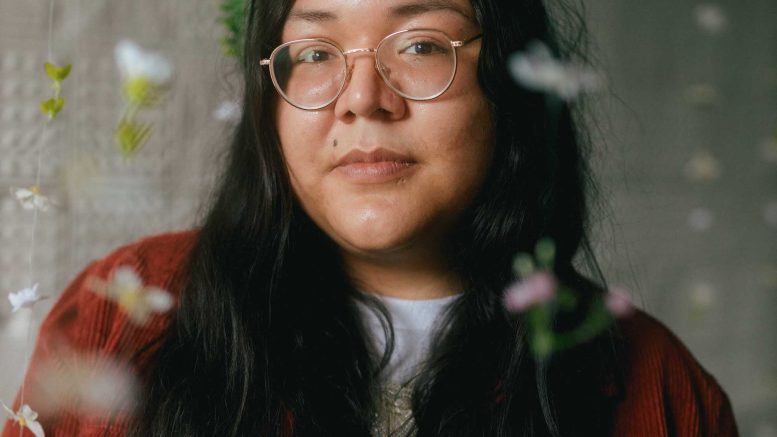This is a close-up image of a young woman, displayed from just above her eyebrows to slightly below her shoulders. She gazes directly into the camera with a neutral, pensive expression, her lips relaxed. The background is a blurry gray-black, with a hint of a green wreath on the wall behind her head that's barely visible. Her long, dark brown to jet-black hair falls past her shoulders, partially concealing the white t-shirt she is wearing. Over the t-shirt, she dons an orange corduroy jacket that gives off a textural contrast. She wears silver metal-rimmed glasses and has a distinctive mole just above her lip on the right side of her face. The background features strings hanging from above, adorned with green and white flowers, framing her figure subtly but distinctively. Her kind, contemplative demeanor is captured in the precise framing and soft background details.